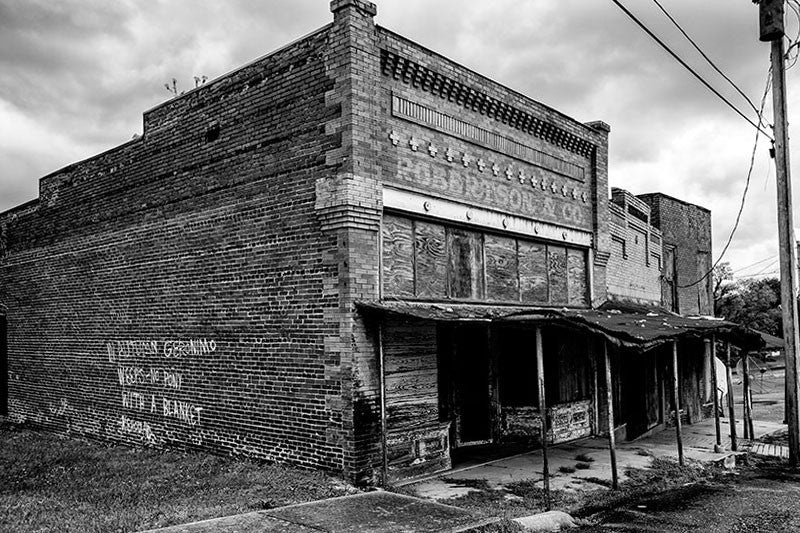The photograph depicts a black-and-white image of an abandoned brick building, likely from the late 1800s or early 1900s. This vintage image showcases a dilapidated storefront with worn, faded signage that reads "Robertson and Company." The storefront has glass display panels and an alcove with rotting doors. The entire structure is in a state of disrepair, with boarded-up windows and a collapsed overhang that once provided cover for a walkway. 

On the left side of the building, the brick wall is adorned with white graffiti, difficult to read but mentioning something about Geronimo, possibly a phrase like "In autumn Geronimo weeps. No pain with a blanket." The graffiti hints at the building's long-abandoned status.

To the right, two additional brick buildings, equally decayed, further emphasize the area’s abandonment. The surrounding environment includes an overgrown concrete walkway, a tall light pole with visible power lines, and an empty lot to the left of the main building. The photo was likely taken on a dark, cloudy day, with a sky filled with clouds, adding to the somber tone of the scene. The image, despite showing a bygone era, is clear in detail and uses natural lighting to highlight the architectural degradation and the atmosphere of neglect.